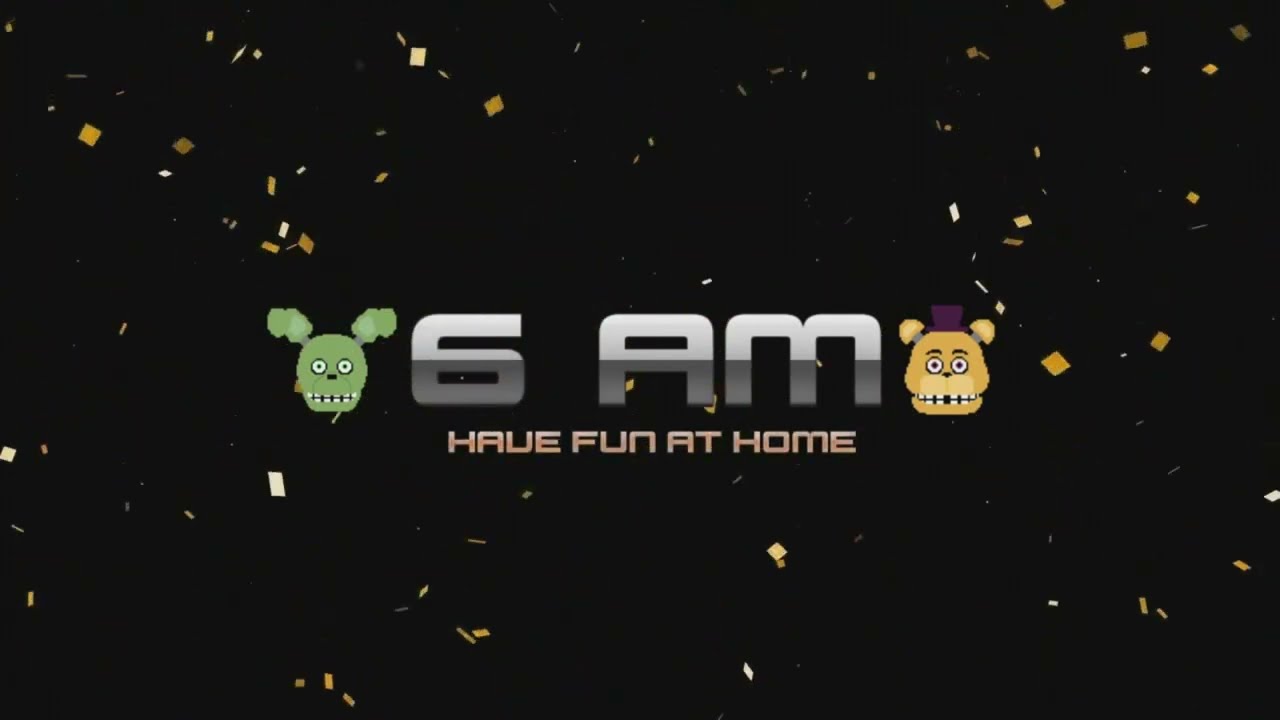This image appears to be a screenshot from a video game, possibly from the "Five Nights at Freddy's" series, given the character design and font style. The scene centers around a large, metallic "6AM" in capital letters, suggesting a moment of victory or transition in the game. Directly below the time, in a smaller copper-colored font, it reads "Have fun at home."

On the left side of the "6AM" text is a green, poodle-like character with foliage-like ears, while on the right side is a teddy bear with a distinctive purple top hat — both displaying the series' signature design of large eyes and somewhat unsettling features. The background is predominantly black, but it is animated with floating gold confetti, enhancing the celebratory feel of the scene. Alongside the black, colors like white, gray, silver, brown, purple, yellow, and green give a vibrant contrast. 

Overall, the arrangement and visual elements suggest that this scene marks a successful completion of a stage, likely after surviving a night in the game, as indicated by the confetti and the message to "Have fun at home."